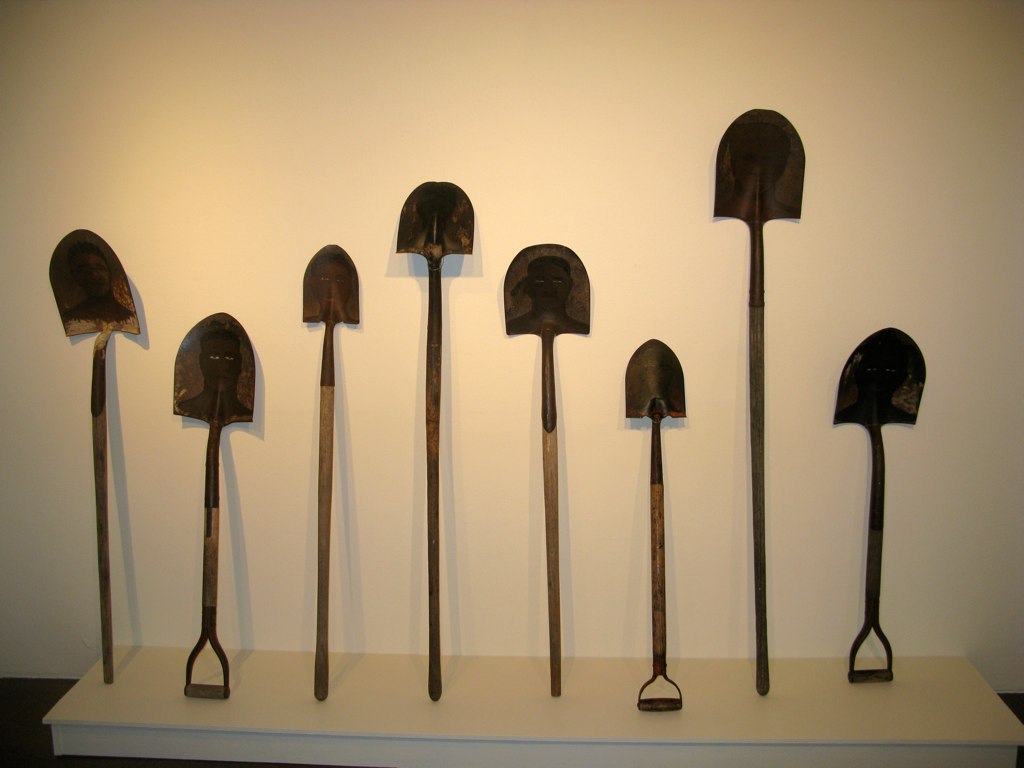In the image, we see a detailed display of eight vintage shovels arranged in a row against a white wall with a black floor. The shovels are positioned standing on their handles with their blades upright on a white shelf system at the bottom. This shelf is raised about two inches off the floor and spans roughly seven feet in width.

The collection showcases a variety of handle lengths and designs. Some shovels feature very long, straight handles, while others have shorter handles with grab handles at the end. Notably, three of the shovels have perpendicular hand grips, distinguishing them as spades. The shovel blades vary in style and condition, from shield-shaped blades with curved tips to more elongated and straight-edged designs. Each shovel exhibits a weathered, rusted brown color indicative of their vintage nature.

Starting from the left, the first shovel is approximately two feet long with a heavily rusted blade. The second shovel is shorter, its handle shaped such that it creates the illusion of a person’s face with eye slits in the rust pattern. This intriguing feature is similarly observed in the next few shovels but becomes less discernible in the subsequent ones. Particularly noteworthy is a small gardening shovel, third from the left, and a large, long-handled digging shovel, second from the right.

Overall, the shovels, characterized by their stained, dark, and weathered appearance, present a fascinating snapshot of utilitarian tools from a bygone era, elegantly displayed on a modest yet effective platform.